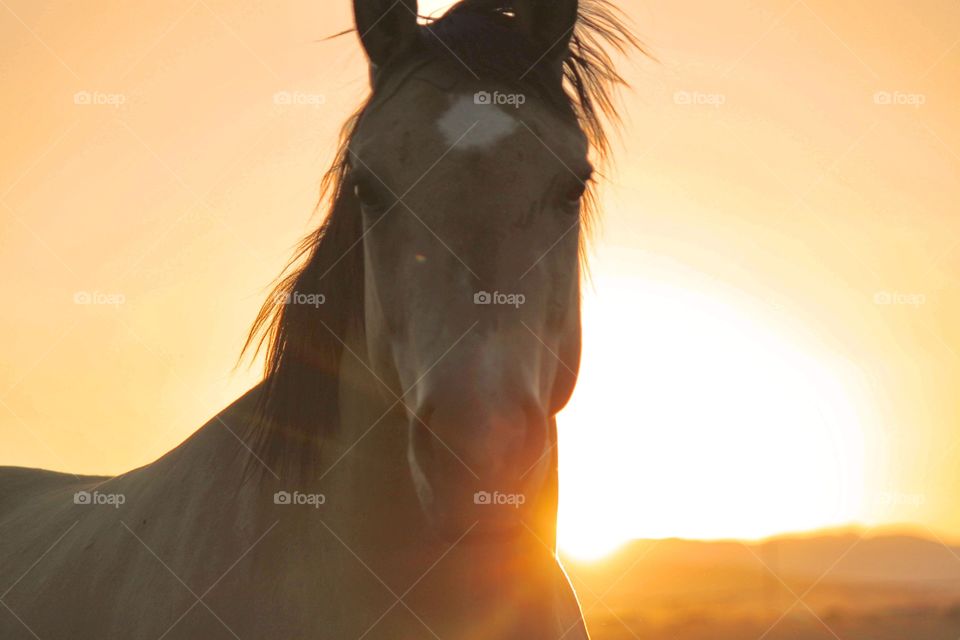The image captures a serene outdoor landscape at either sunrise or sunset. Dominating the scene is a horse positioned towards the bottom left, slightly off-center, with its body extending upward towards the center of the photograph. The horse's head is prominently featured, facing directly at the camera. Its coat is grey, complemented by a black mane and black eyes, and it has a distinctive white star on its forehead. The sun, bright yellow and almost white, is nestled next to the horse's neck, creating a striking contrast with the surrounding sky, which fades through shades of orange, yellow, and brown. A landscape feature is subtly visible in the bottom right corner, casting darker hues of orange and brown. The entire image carries a faint watermark that reads "FOAP" along with a delicate crisscross pattern, indicating it might be a stock photo. The colors blend harmoniously, presenting a vivid interplay of natural light and the tranquil presence of the horse, suggesting a farm setting.